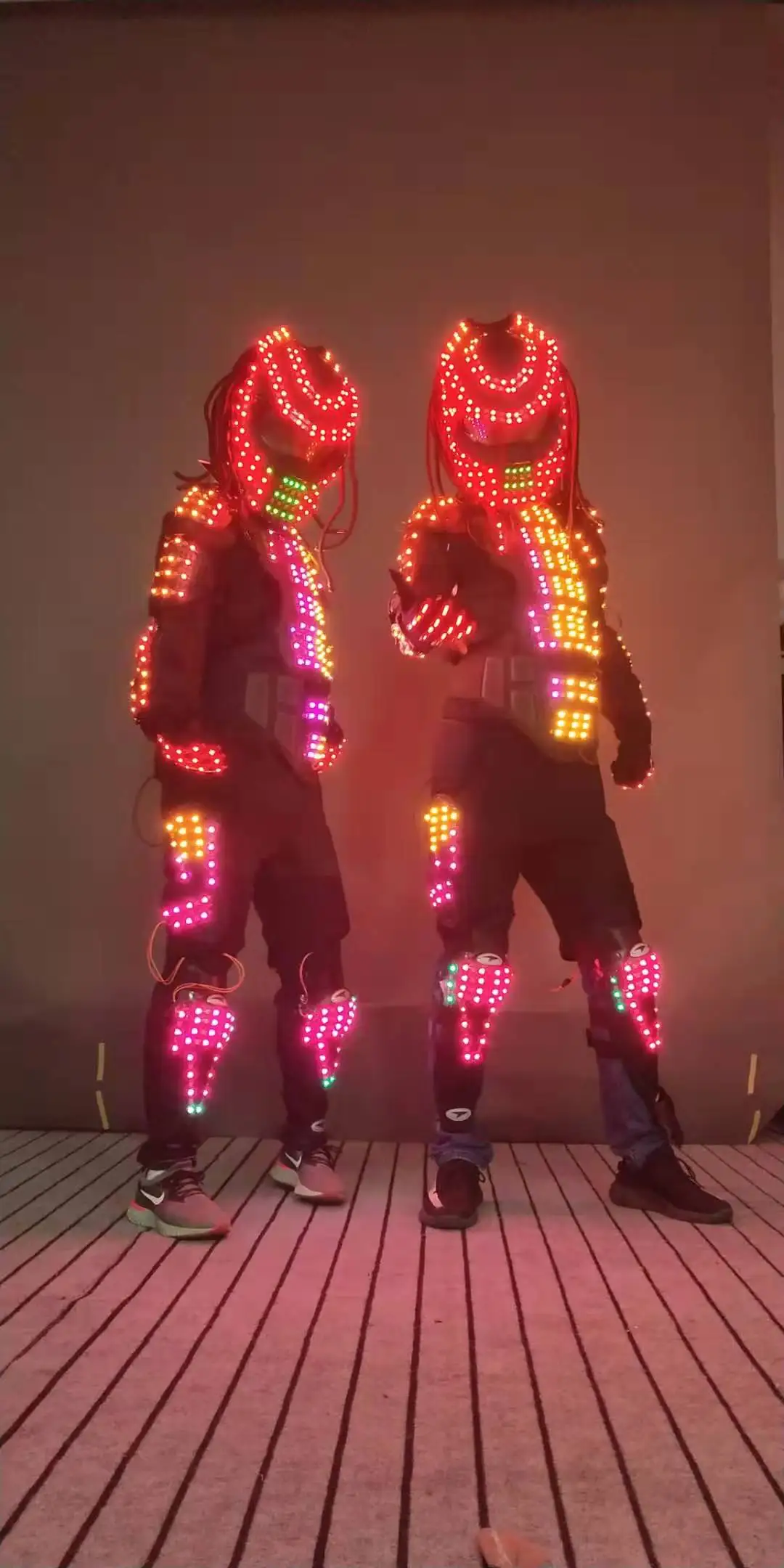This image captures two individuals standing side by side on a wooden deck against a reddish-brown wall, both wearing identical costumes illuminated with vibrant LEDs. The base of their costumes is black, and each is adorned with intricate LED patterns. Their masks, reminiscent of the alien from "Predator," feature glowing red lights circling the top and extending down the face, with three rows of green lights at the mouth. Their dark shirts are decorated with pinkish-red lights down the chest and orange lights on the right arms, composed of three rectangular yellow-lit boxes. The pants have yellow and pink accents, particularly around the knees and where cargo pockets would be, with further LED embellishments on the thighs. Each person is wearing tennis shoes, one notably a pair of Nikes, and the individual on the right has a glowing red glove and extends an arm outward as if pointing at the camera.